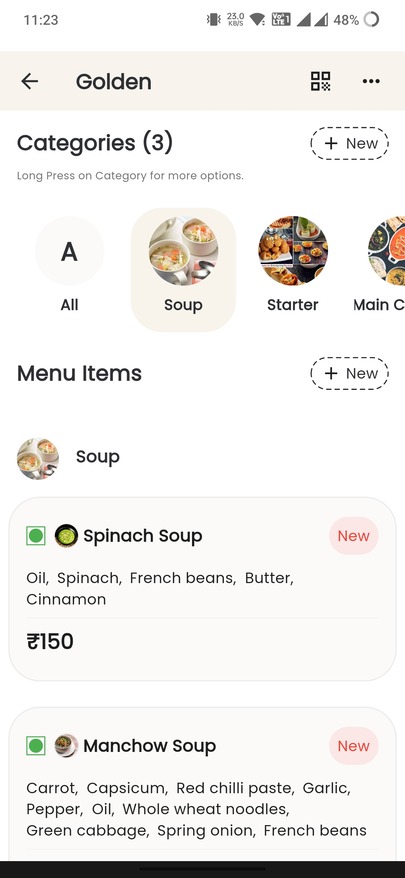A detailed caption for the image based on the provided description could be:

"This color screenshot shows a food-related application on a smartphone at 11:23 AM with a battery life of 48%. The phone has a strong network connection. The app's name isn't visible, but the user is on the 'Golden Section' screen. Below the section title, there are three categories: Soup, Starter, and Main Course, with the user currently hovering over the 'Soup' option. This action reveals two menu items: Spinach Soup, made from oil, spinach, French beans, butter, and cinnamon, and Carrot Mancho Soup, containing carrot, capsicum, red chili paste, garlic, pepper, oil, whole wheat noodles, green cabbage, spring onion, and French beans. The prices for these soups are displayed in an unfamiliar currency, possibly Korean."